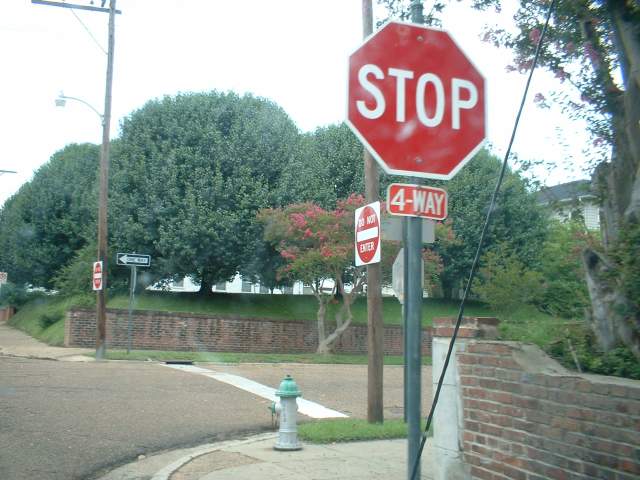This image depicts a street corner at a four-way intersection, dominated by a prominent red stop sign with a white "FOUR-WAY" label affixed beneath it. Adjacent to the stop sign is a white and bluish-green fire hydrant, positioned in front of a wooden pole displaying a "DO NOT ENTER" sign. The street markings include a solid, bright white line, indicating the crosswalk. 

Behind the stop sign, a partially crumbling brick wall stretches along the sidewalk, with a densely foliaged area that includes large, unmanicured trees and others adorned with red flowers. 

Across the street on the opposite corner, another "DO NOT ENTER" sign can be observed, mounted on a light pole, alongside a black and white one-way sign directing traffic to the left. Additional features include a continuous brick wall lining the opposite side of the street, obscuring a white building, possibly residential or office space, shrouded by manicured, green trees. The atmosphere appears bright but overcast, with a white sky suggesting cloudy weather. The scene evokes a mix of aged infrastructure with evident signs of wear and natural greenery that varies in maintenance level.